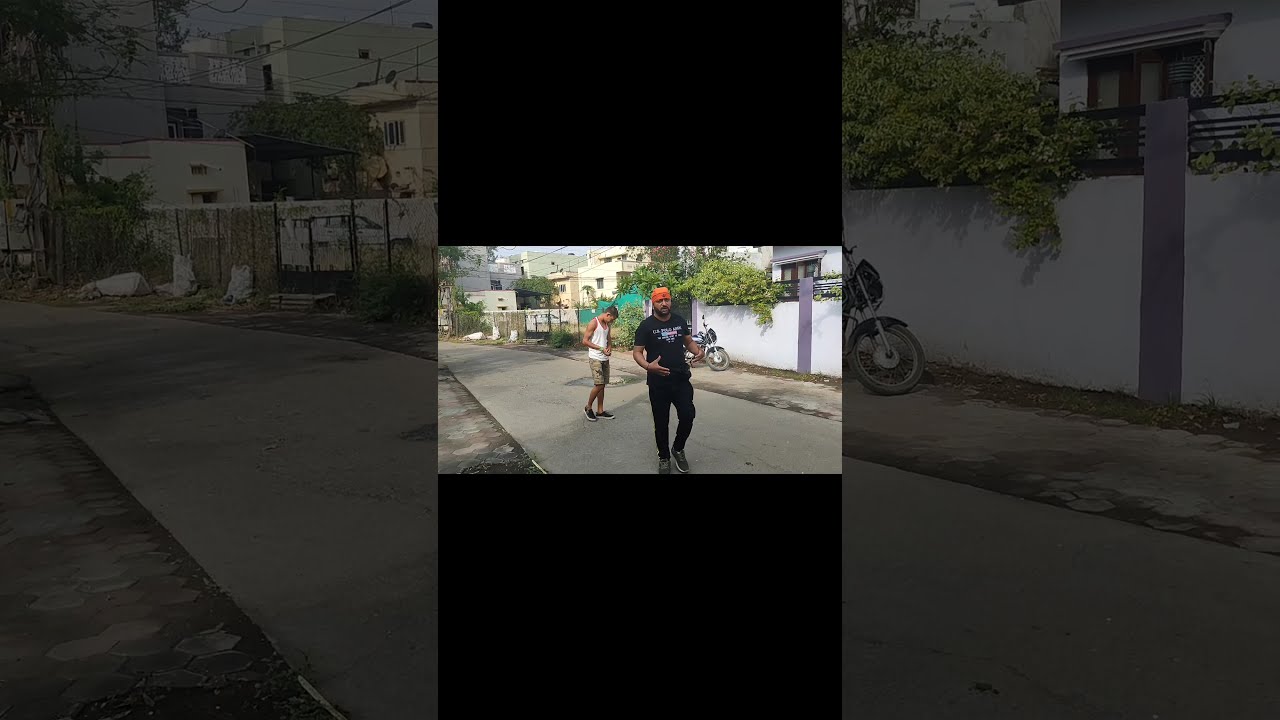This photograph, likely a still from a TikTok video, depicts two men walking on a residential street. The primary subject, positioned in the foreground and slightly to the right, is a black man dressed in a black t-shirt, black pants, and gray sneakers, with an orange do-rag wrapped around his head. He sports a black beard and appears to be looking towards the camera. Behind him, to the left, is another black man who seems younger. He is wearing a white sleeveless tank top, khaki shorts, and dark shoes, and is looking downwards. In the background, partially obscured, is a motorcycle leaning away from the viewer. The setting includes beige buildings with white fencing and some purple columns, stone pathways, worn areas of the road, and visible electrical lines overhead. The image itself sits center within a larger, darker frame made up of enlarged, grayed-out portions of the same photo, creating wide borders on all sides and emphasizing the focal point in the middle.